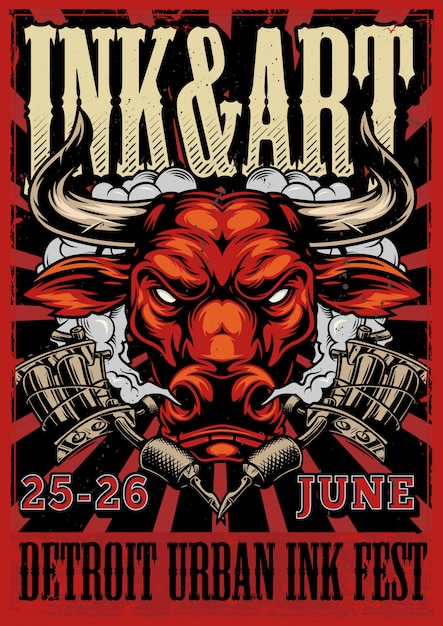This poster advertises the "Detroit Urban Ink Fest," a tattoo festival. The main background color is red, accentuated by black rays emanating from behind a fierce brown bull in the center. The bull has prominent white horns, red ears, and angry white eyes, with smoke billowing from its nostrils. Above the bull, in large light yellow letters, the words "Ink and Art" are prominently displayed. Flanking the bull on both sides are tattoo guns with their needles crossing in front of its face. The dates of the festival, "June 25th - 26th," appear below the tattoo guns in red letters outlined in white, with all details culminating in the bold black text at the bottom declaring "Detroit Urban Ink Fest."